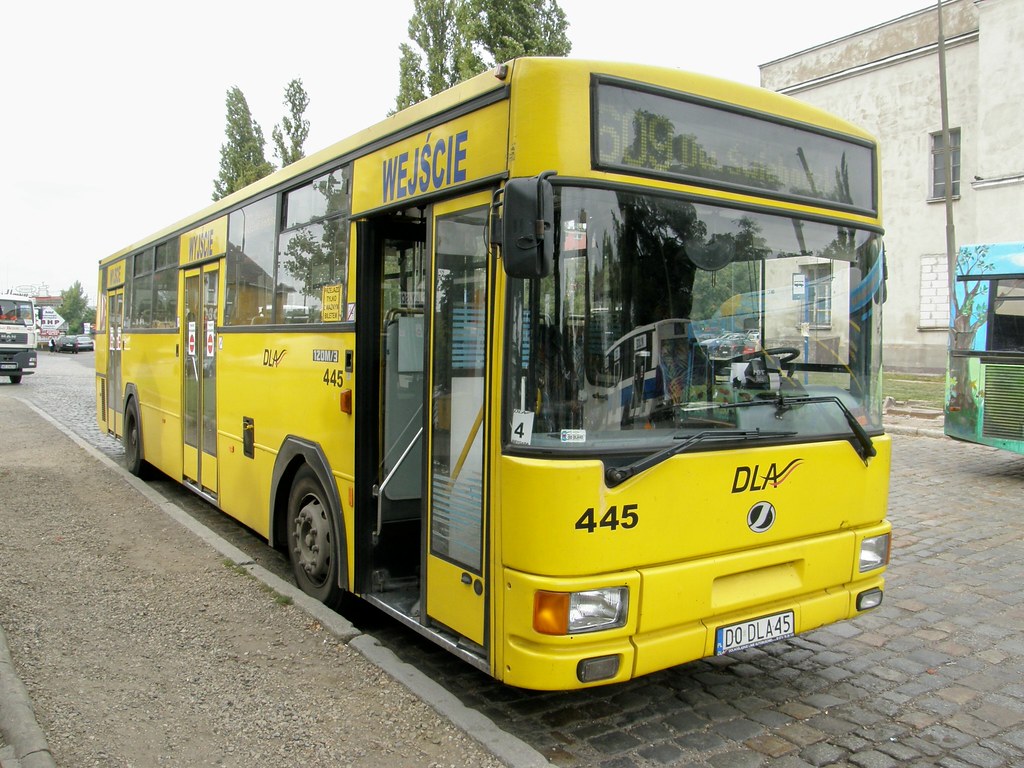This image displays a large, bright yellow European city bus, parked on a narrow, cobblestone street alongside a light brown, gravel-coated sidewalk. The bus, which appears modern and well-maintained, has a prominent electronic sign at the top indicating its route, "609 Dishwise Bosque," though the exact spelling is unclear due to glare. The bus features three sets of double doors along its right side, designated for passenger entry and exit. Above each door is the word "WEJŚCIE," likely indicating "entry" in a language such as Polish. The bus is marked with the identifiers "DLA" and "445" at its front, along with a license plate that reads "D0 DLA 45," which resembles a European format. The front door is open, ready to admit passengers, but no driver is visible due to the glare on the windshield. Surrounding the bus are parked vehicles, a cream-colored building, and the tops of trees emerging in the background, which contribute to the setting's urban landscape.